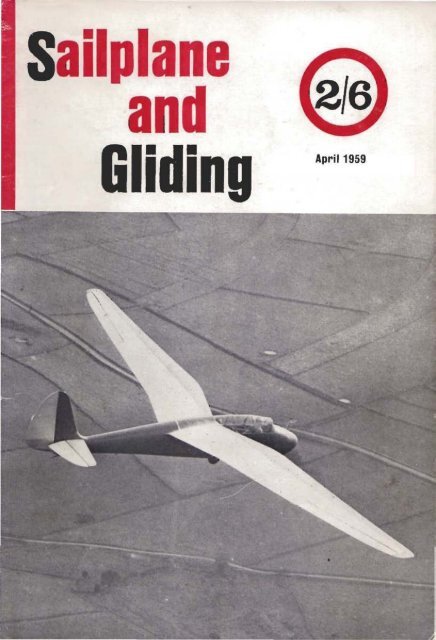The image appears to be the cover of a vintage magazine titled "Sailplane and Gliding" from April 1959. The magazine's title is prominently displayed in a large, white banner at the top of the cover, with the text in bold red and black letters. To the right of the title, the issue number "2-6" is indicated in black numerals inside a red circle, likely signifying it as the second of six issues for the year. The photograph that occupies the rest of the cover is in black and white, showing a glider aircraft soaring high above a patchwork of farmland below. The land is sectioned into geometric plots and roads typical of agricultural areas, all rendered in varying shades of gray due to the monochromatic nature of the image. The glider itself is characterized by its simple design, featuring long wings and a tail wing, and appears to lack any visible engines, emphasizing its nature as a sailplane. One of the wheels is faintly visible beneath the aircraft. Overall, the cover exudes a distinctly vintage aesthetic, capturing a moment in aviation history from the late 1950s.